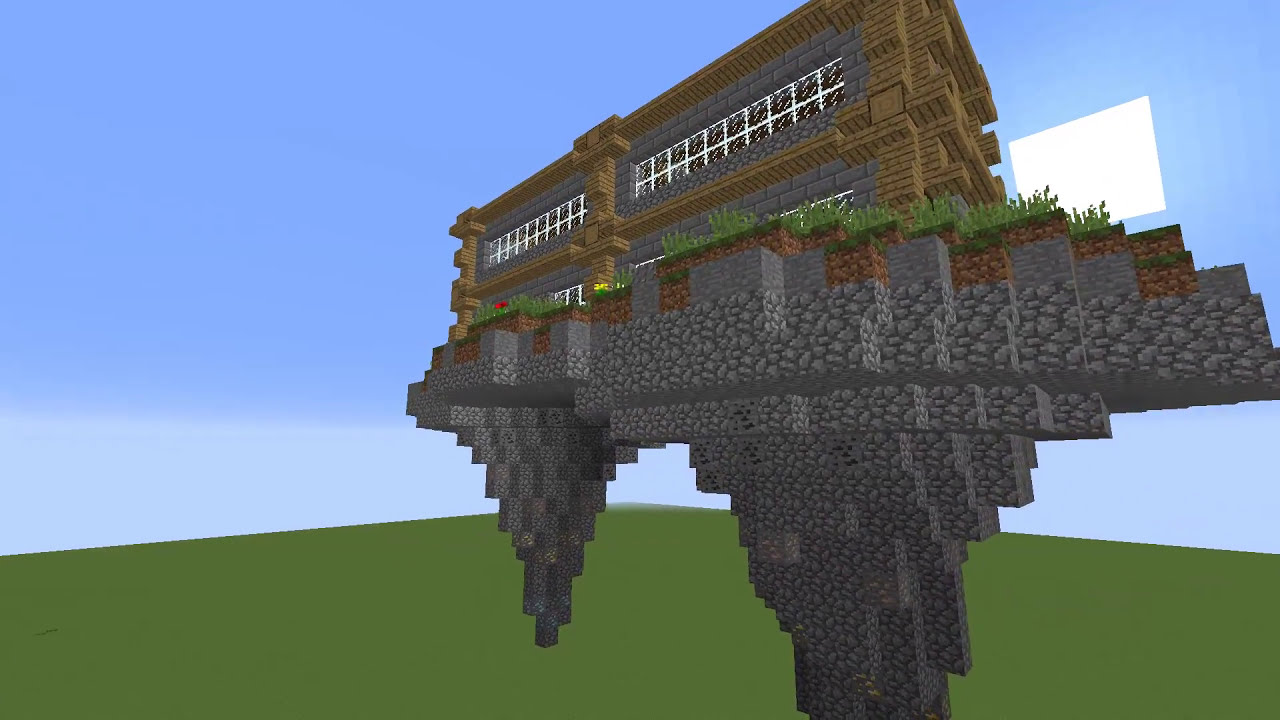In this pixelated digital creation, likely a screenshot from a video game resembling Minecraft, a horizontally oriented building hovers in the air. The scene is vividly colored with a bright blue sky occupying the upper half, underlined by a faint white strip. Below, there's a stretch of plain green grass. The floating structure is supported by two asymmetrical pillars on either side—both constructed from various shades of gray stone.
 
The left pillar is slightly off-centered to the left, while the right pillar dominates the bottom right corner of the image. Atop these pillars rests the main building, which features a brown wood exterior interspersed with gray stone sections. The building has two horizontal windows bordered in black and white. Surrounding the building, there's a mix of lighter green grass and patches of red and yellow flowers. The structure appears to float above a forest-green base, connecting its earthy tones to its environment.